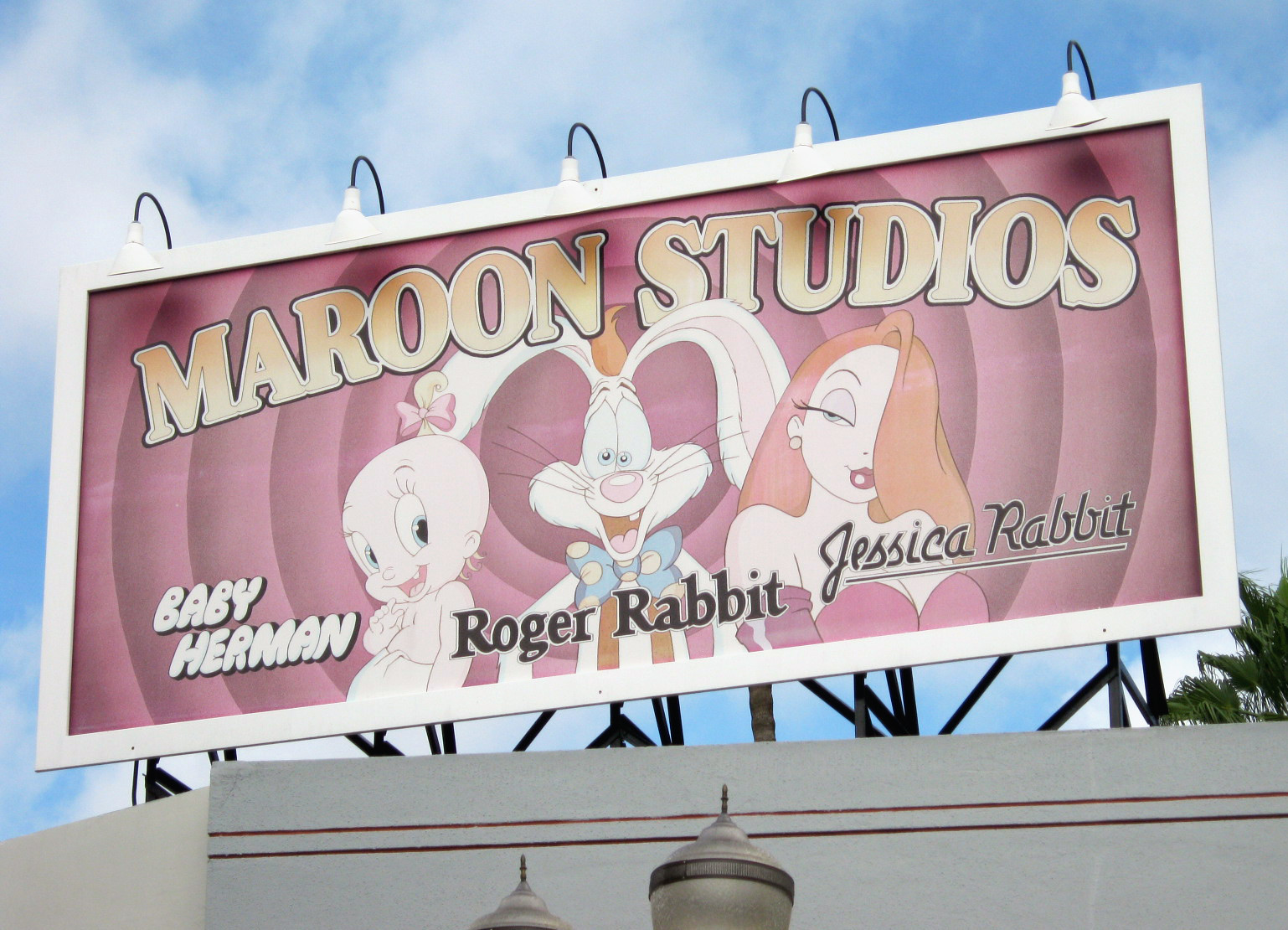In this landscape-oriented color photograph, we see a large billboard mounted on top of a white building adorned with light and dark maroon stripes. The clear blue sky, dotted with thin, foggy-looking clouds, serves as the backdrop while green palm leaves peek over the building’s roof. The bottom edge of the image captures the tops of streetlights.

The billboard, framed in white, showcases five white spotlights arched over its top, ready to illuminate the display during nighttime. The visually striking billboard features concentric radial circles ranging from pink to purple, reminiscent of the iconic Looney Tunes spirals. At the top, bold gray-gold gradient letters spell out "Maroon Studios" in a slight curve.

Standing out prominently on the billboard are three cartoon characters: Baby Herman on the left, Roger Rabbit in the center, and Jessica Rabbit on the right, with each name labeled accordingly. Baby Herman is depicted with a pink bow in her hair, Roger Rabbit exudes his usual quirky charm, and Jessica Rabbit stuns in her signature red outfit. This image epitomizes photographic representational realism, capturing a vivid and detailed portrayal of the scene.